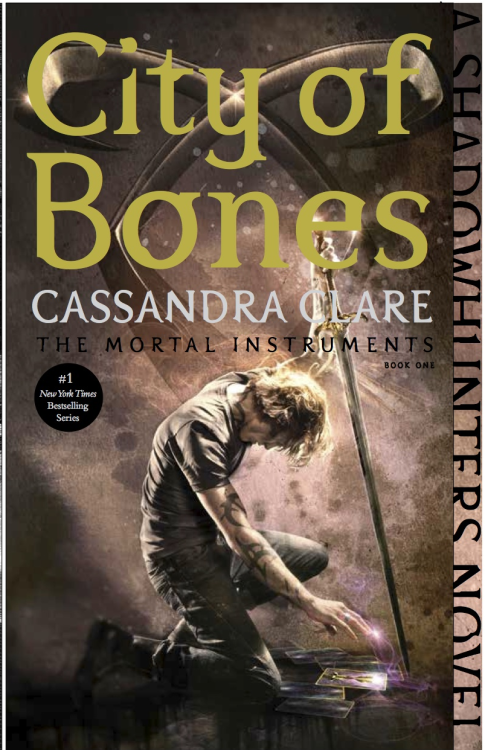The image is a vertical rectangular book cover predominantly brown with lighter shades integrated. At the top, in large gold letters, it says "City of Bones," with "City" and "Bones" capitalized. Just below the title, in white, capitalized text, is the author's name: Cassandra Clare. Underneath that, in black letters, it states "The Mortal Instruments" followed by "Book One." A black circle on the left side announces "Number One New York Times Bestselling Series" in white font. On the right side of the cover, written vertically, it reads "A Shadowhunter Novel."

The central illustration depicts a man kneeling, with electricity or light emanating from his right fingers. He seems to be interacting with pictures or symbols on the ground. He is holding a staff or weapon, possibly a scythe, and wears a short-sleeved shirt that reveals tattoos on his right arm. The scene has a dark, fantastical ambiance with beige and pink undertones, suggesting a sci-fi or fantasy realm.